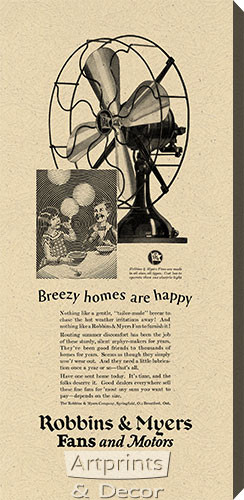The image appears to be a vintage advertisement, intentionally designed to look aged, featuring a beige-colored background. Central to the image is an antique fan with metal wires across the front, evoking a sense of nostalgia. Below the fan, there is a charming black and white photograph of a young girl and a man, seated together at a table with three large, balloon-like objects floating above them. The text, although blurry and hard to read, includes the prominent phrase "Breezy Homes are Happy" in a serif font. At the bottom, it clearly states "Robbins and Meyers, Fans and Motors," followed by "Art Prints and Decor." The overall composition suggests a blend of functionality and artistic appeal, characteristic of old-time promotional material.